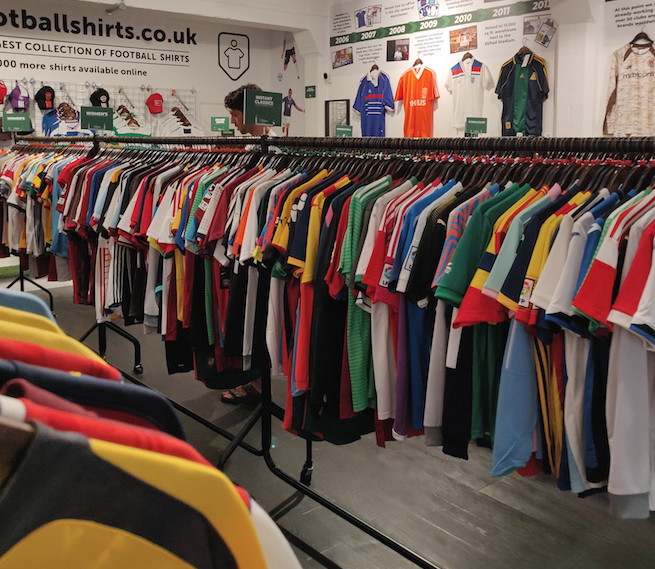The photograph captures the vibrant interior of a British store specializing in soccer jerseys, branded footballshirts.co.uk. Dominating the center of the image is a long rack filled with a vivid array of football shirts, featuring a kaleidoscope of colors such as blue, yellow, red, green, white, and black, with about 50 to 75 shirts neatly hung. The backdrop is a dark brown wooden floor that adds a touch of warmth to the scene. The back wall prominently displays the store’s name and slogan, "footballshirts.co.uk - Best collection of football shirts. More shirts available online." This wall, along with another perpendicular wall to the right, showcases jerseys organized chronologically by dates, such as 2006 and 2007, creating a visual timeline of football fashion. Additional shirts and hats are also hung on these walls, echoing the diverse palette seen in the center rack. Tucked away in the left-hand corner of the image is another partial rack, peeking into the frame with more vibrantly colored shirts, including yellow and black, red, brown, blue, and orange. This detailed depiction underlines the extensive variety and dynamic presentation of football apparel offered by the store.